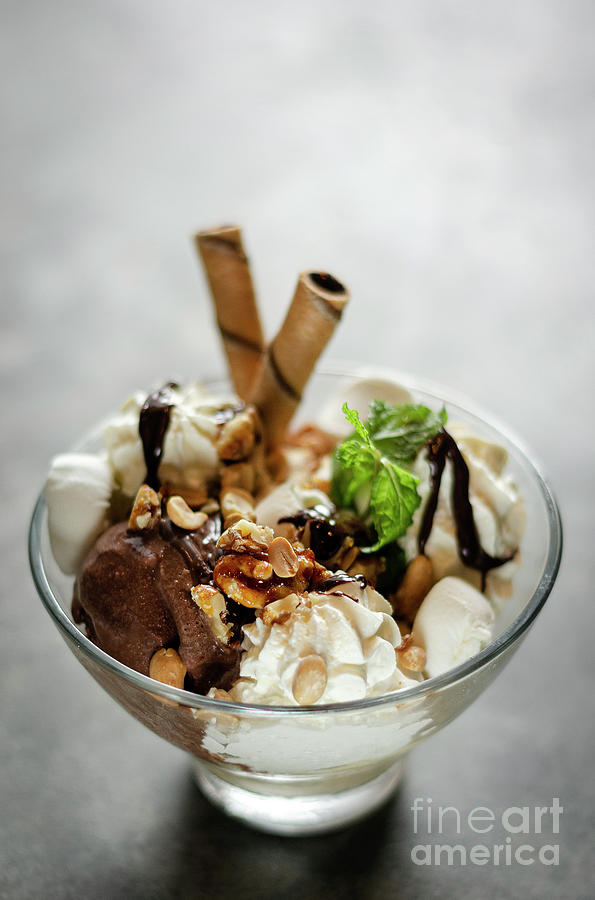This photograph features a sumptuous ice cream sundae presented in a clear glass bowl, resting on a gray table against a blurred gray background. The bottom right corner of the image displays the text "Fine Art America," with "Fine" in a thin font and "Art America" in bold white letters. The sundae itself is an indulgent mix of what appears to be vanilla and chocolate ice cream, generously topped with whipped cream, a rich hot fudge sauce, and crunchy peanuts primarily scattered toward the front of the bowl. Adding a refreshing touch, a sprig of green mint is nestled at the center of the dessert. Also adorning the sundae are two tube-shaped, chocolate-filled dessert sticks, artistically placed upright in the back. The overall presentation promises a delightful blend of textures and flavors, making it a feast for both the eyes and the palate.